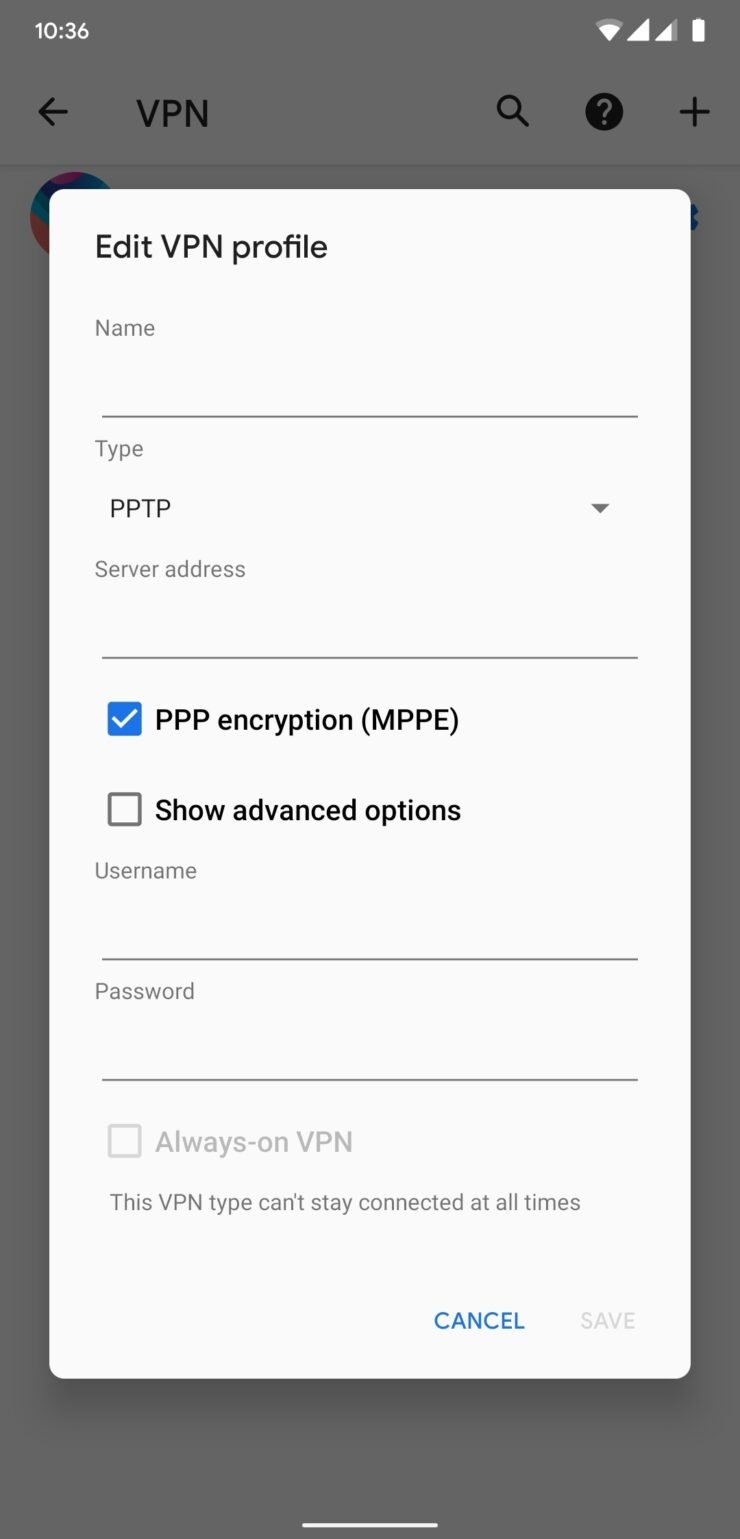A detailed screenshot of a cell phone display is captured at 10:36, either a.m. or p.m., as indicated by the clock at the top of the screen. The battery icon in the upper right corner shows a full charge. Also located in the upper right corner are two different signal strength indicators: one indicating full strength with four bars, and another showing a slightly weaker signal with three out of four bars. The presence of a Wi-Fi connection is denoted by an upside-down triangle symbol filled partially to represent moderate signal strength. Additionally, a VPN status is visible next to the Wi-Fi indicator.

At the top of the screen beneath the signal indicators is a navigation bar, including a back arrow on the left side and a search bar in the center, containing the text "VPN" and a magnifying glass icon on the right end. Alongside the search bar, there is a black circle housing a white question mark, followed by a plus sign likely meant for adding a new VPN profile.

Central to the screenshot is a pop-up within the app displaying the word "edit," suggesting an option or mode for modifying settings or content.